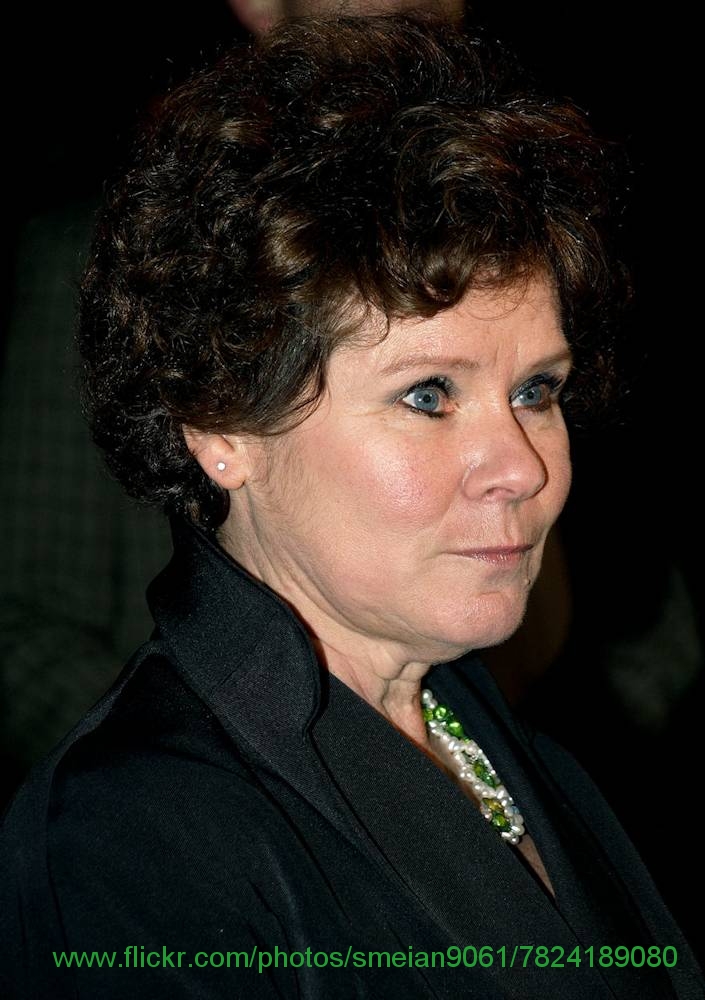This photograph captures a middle-aged to older woman with expressive, very light blue eyes accentuated by eyeliner and done-up eyelashes. She is adorned in a black jacket, under which a striking necklace of white pearls and emerald-green jewels sparkles around her neck. Her short, curly dark brown hair frames her face, and a single stud earring—a small diamond or pearl—glistens in her ear. She gazes off to the right, her expression neutral yet tinged with a hint of a restrained smile. The backdrop is dark and blurred, with just a glimpse of a plaid-patterned shirt suggesting the presence of another person in the obscured background. The URL "www.flickr.com/photos/smian9061/7824189080" is inscribed in green text at the bottom of the image, which is clearly focused on her.